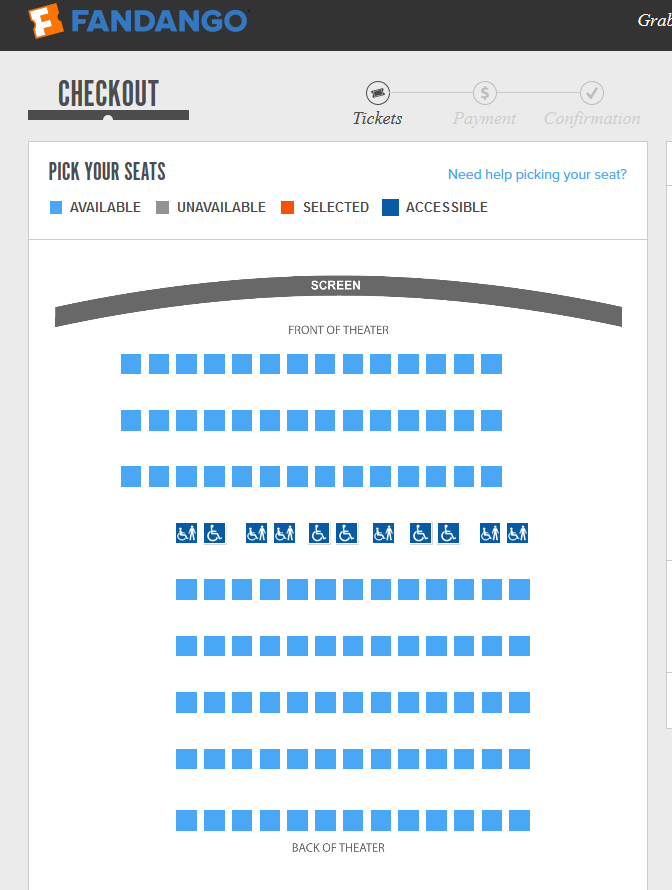A screenshot of the Fandango website displays various elements prominently. At the upper left-hand corner, "FANDANGO" is presented in bold, all-capital letters with a blue font. Adjacent to the left, the Fandango logo features a white "F" embedded within an orange ticket-shaped silhouette.

Beneath this, the interface highlights the current stage as "CHECKOUT," indicated by grey capital letters with an underscore. To the right, a progress bar illustrates the steps: "Select Tickets," "Payment," and "Confirmation." The screen is currently on the "Pick Your Seats" stage.

Directly under "Pick Your Seats," a color-coded legend clarifies the seating options: blue denotes available seats, grey indicates unavailable seats, orange signifies selected seats, and dark blue shows accessible seats. Below the legend, there is a detailed layout of rows of chairs representing the movie theater seating arrangement.